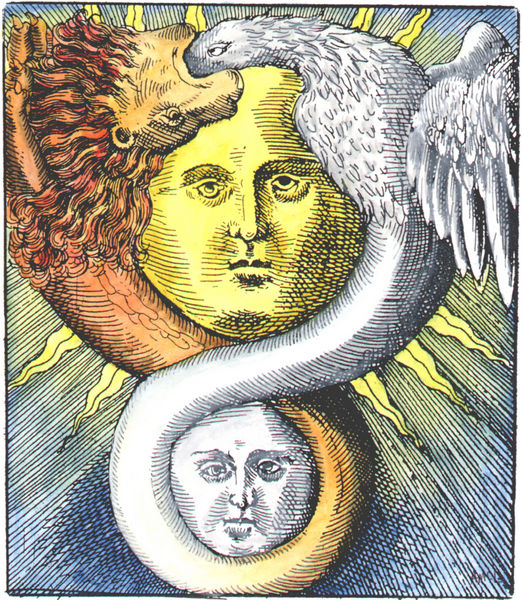This artwork is a vertically-oriented drawing, primarily made with pen or pencil and accented with colored pencils. Dominating the composition are two prominent round faces arranged vertically. The top face, resembling a radiant yellow sun, stares intently at the viewer, emitting sun rays. Below it is a smaller, grayish-white moon face with similarly expressive features.

An abstract creature intertwines through the image. On the left side, the creature starts with an upside-down lion's head, colored brownish-orange, which is seen devouring the face of a white eagle. This lion transitions into a snake-like body that wraps around the moon face, eventually merging into the form of the eagle. The creature’s body forms a continuous loop, creating an almost yin-yang visual effect. The background is filled with a blue hue, adding depth to this surreal and intricate scene. Numerous lines and abstract patterns weave throughout the image, enhancing its complex and odd appearance.